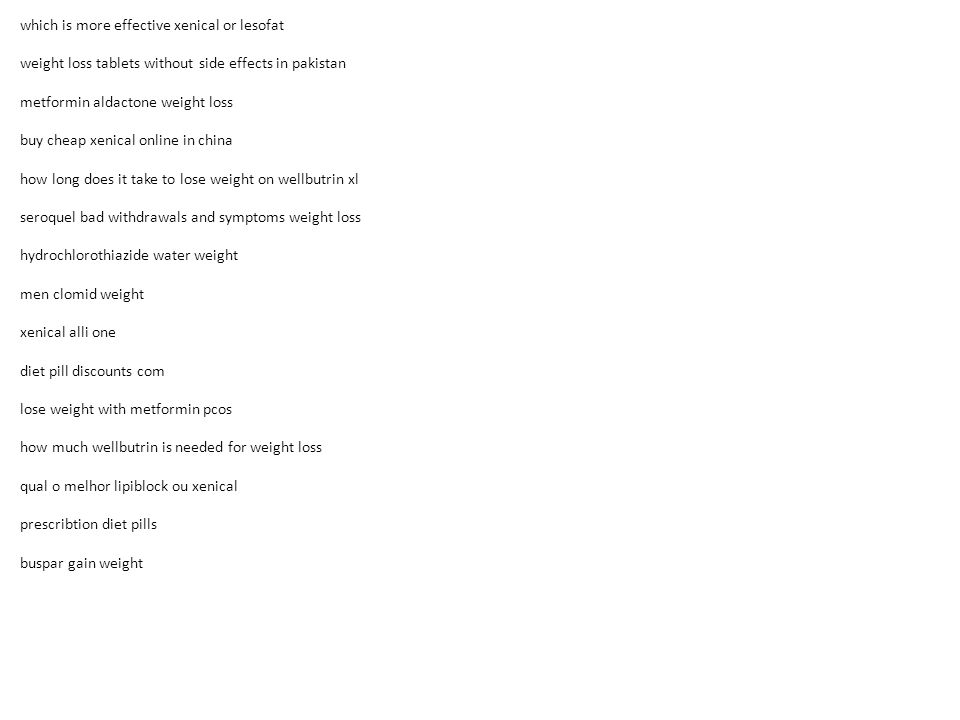The image appears to be a screenshot of a text-only webpage with a plain white background. The content is a serious and straightforward list of weight loss-related topics and products, with the first line reading: "Which is more effective, ExeCal or WesoFet? Weight loss tablets without side effects in Pakistan." Additional terms and phrases scattered throughout the text include "Melatonin," "Atatone weight loss," "BuyCheap ExeCal online in China," "how long does it take to lose weight on Wellbutrin," "Cerecal hydrodrols and symptoms weight loss," and "Hydrochloroside water weight." Other mentions encompass "manoclomid weight," "Xenol Alley1," "dietpilldiscounts.com," "lose weight with metformin," "Prox," and "how much Wellbutrin is needed for weight loss." Specific product names like "Qualome for lipid block" and "OU Xenical prescription diet pills" are also noted, alongside a bit about "bulk gain weight." The page is entirely devoid of any images or colors, presenting a stark, monochromatic layout focused purely on the information.